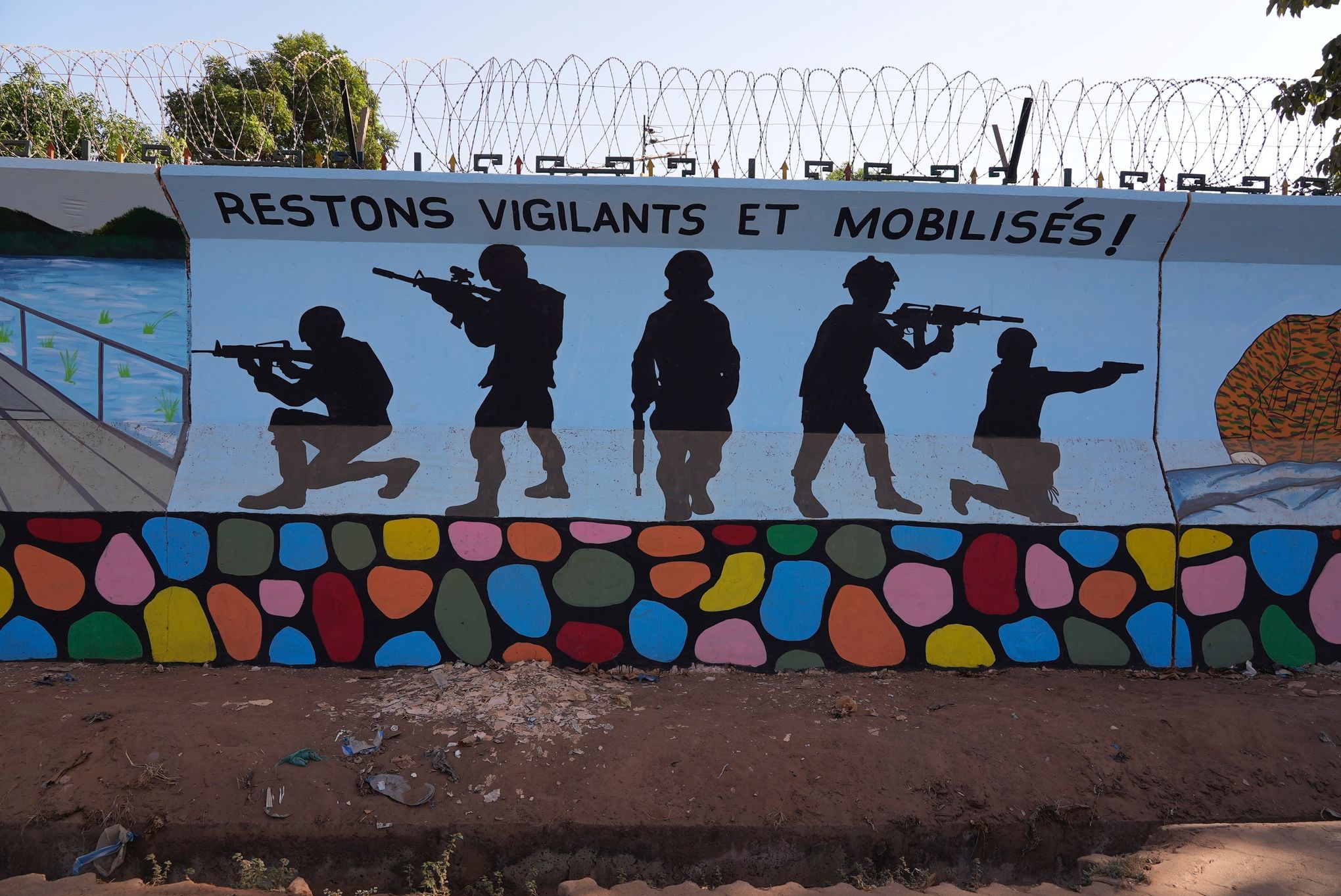This photograph captures a detailed and vibrant mural painted on a white concrete wall topped with barbed wire. In the background, a clear blue sky and the green leaves of two tree tops frame the scene. The mural features a soldier-themed artwork titled "Ruston's Vigilantes at Mobile's," and is set against a light blue backdrop. The composition includes five black silhouettes of soldiers: starting from the left, the first soldier is kneeling and looking to the left with a rifle; next to him, another soldier stands and looks to the left, also with a rifle. The middle figure faces forward holding a rifle to his side, followed by a soldier to his right, standing and aiming his rifle to the right. On the far right, the fifth soldier is kneeling with a pistol, also pointing to the right. Below these figures, a section of the mural mimics a rock wall with variously colored stones in pink, blue, gray, red, yellow, and orange, all depicted with black mortar. The lower edge of the mural shows peeling paint in shades of dark and light brown. Parts of other murals are visible on both the left and right sides of the central image, including a cutoff depiction of a man in camouflage on the right and an image of a bridge over water with mountains on the left, hinting at a larger, interconnected mural theme.